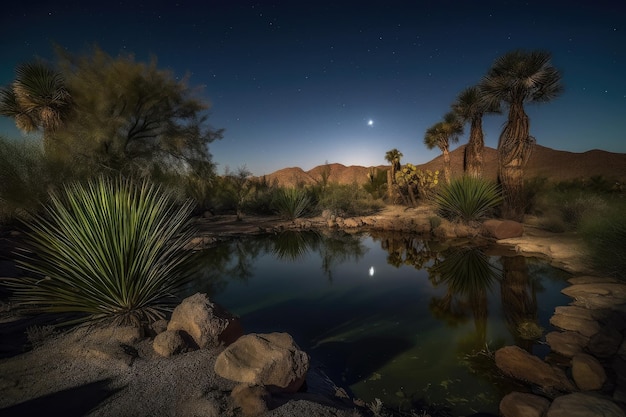This captivating nighttime scene from the southwestern U.S., quite likely Southern California or Arizona, features a serene desert landscape under a dark, star-studded sky. At the center of the image is a small, shallow pond, possibly a desert spring, reflecting the soft light of a shining moon. The moonlight also casts reflections of the surrounding scenery in the water. Surrounding the pond are numerous rocks and rock formations, adding texture to the tranquil scene. In the background, a variety of desert flora can be seen, including Joshua trees, yucca plants, cacti, and some palm trees. Notable features include sand hills and low-lying brownish mountains towards the right, and a large, prominent tree on the left. The stark shadows in the foreground add a sense of mystery and depth, contributing to the overall beauty and peace of this twilight snapshot of the Mojave Desert.